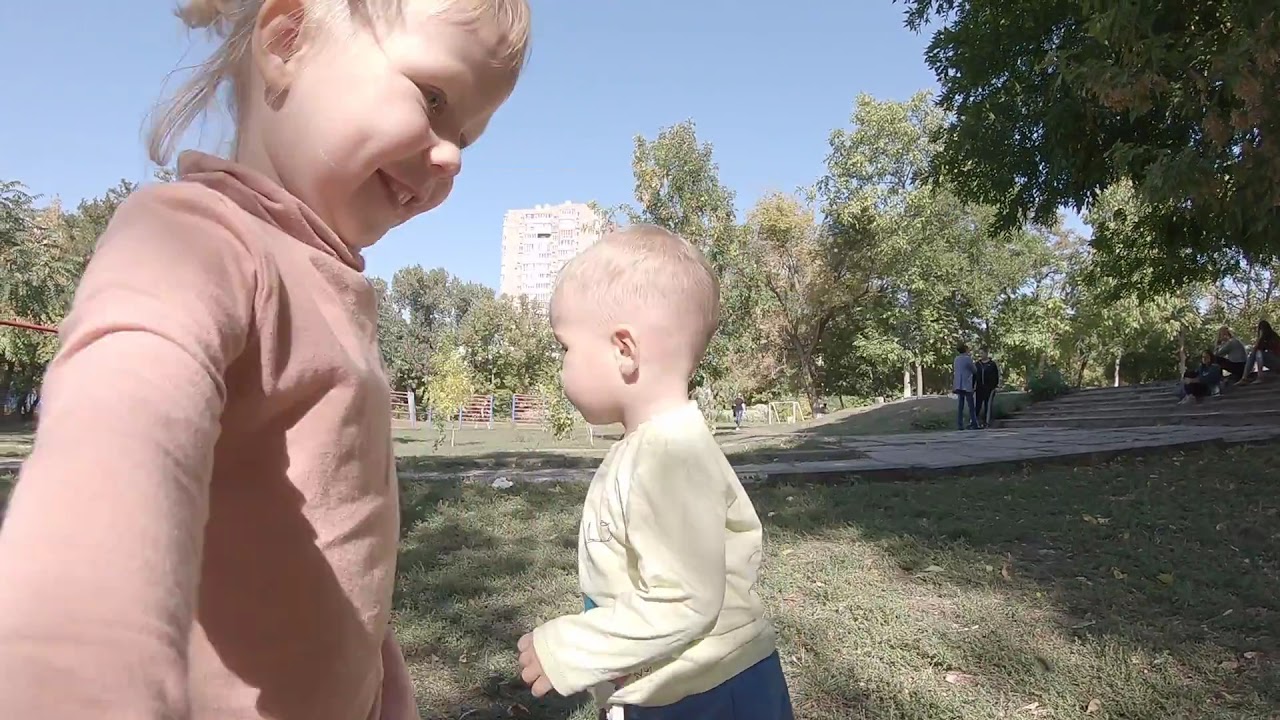The photograph captures a vibrant park scene on a clear, sunny day. The sky is a light blue without a cloud in sight, providing a serene backdrop for the multi-story residential building that stands prominently towards the top center of the image. In the foreground, two small children are the focal point. On the left, a young girl with a cheerful demeanor is wearing a long-sleeve pink shirt. Beside her, to the right, is a younger boy dressed in a long-sleeve yellow shirt paired with blue shorts that feature a distinct white stripe on the side. Both children are standing on lush, green grass.

Further into the image, a cement pathway cuts through the center, leading the eye towards more activity. Standing on the pathway are two older adults engaged in conversation. The adult on the left sports a gray jacket and blue jeans, while the one on the right is attired in a black jacket with matching black pants that have a white stripe. The park also features small trees scattered around, adding to the natural ambiance. People can be seen in various areas of the park, some sitting and some standing, enjoying the sunny weather. The image exudes a lively, communal atmosphere with layers of detail inviting the viewer to explore the scene.